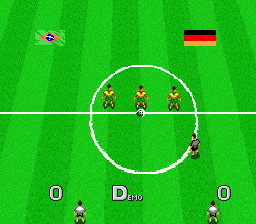This detailed in-game screenshot captures a moment before a soccer match begins in an older, somewhat blocky, soccer-themed video game. The setting features a green, striped field with a prominent white horizontal line and circle at the center. Within this circle, a soccer ball is positioned, ready for the kickoff. At the top left corner, the Brazilian flag is displayed, while the top right corner features the German flag, indicating a match between Brazil and Germany. The top half of the field shows three Brazilian players wearing yellow jerseys and green shorts, positioned at the upper part of the circle. On the bottom half of the field, three German players, wearing white shirts and black shorts, are spaced out below the circle. The bottom of the screen shows a score of 0-0, with "demo" labeled in the center. The overall scene suggests the game is about to commence, with players from each team poised for action.